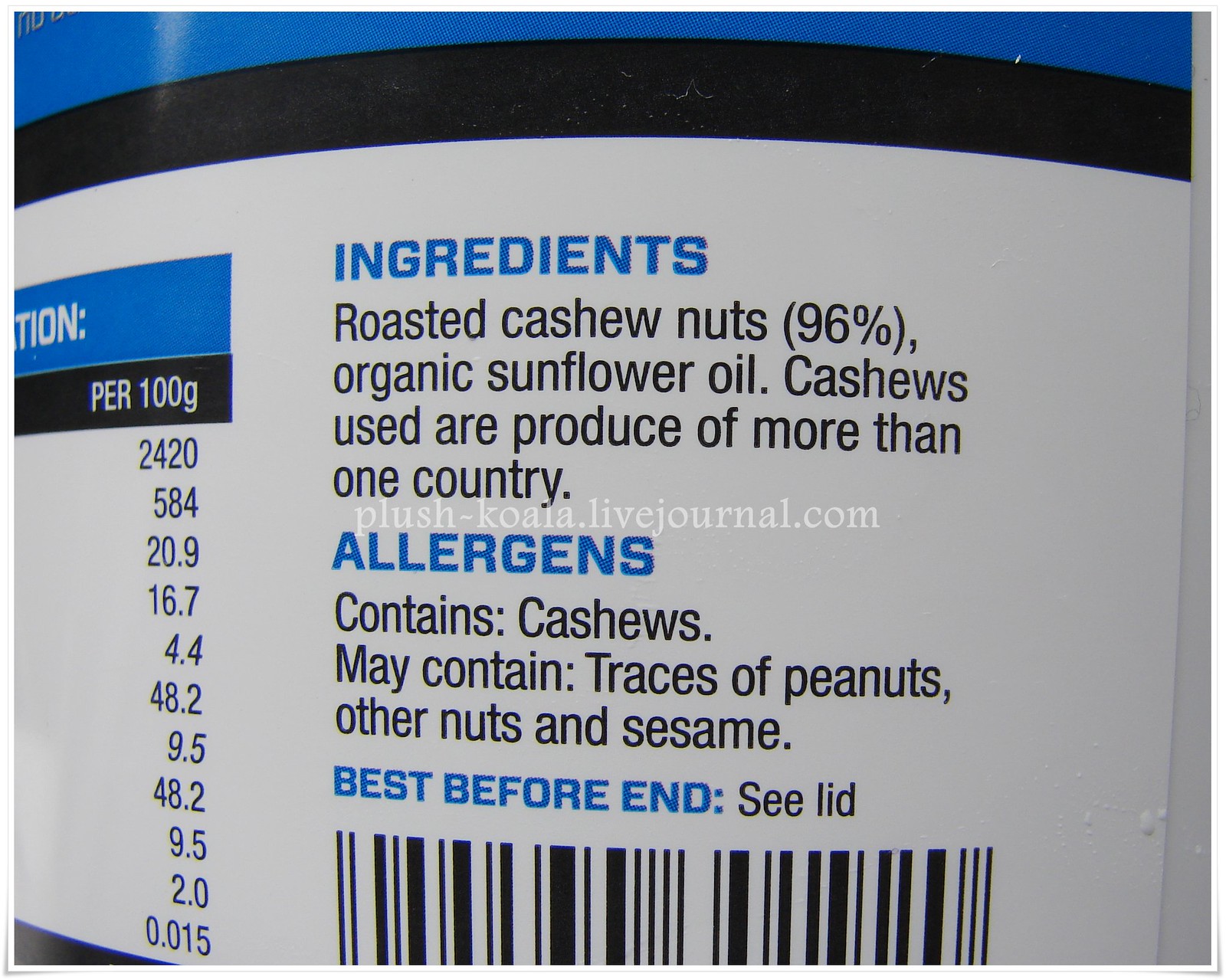This is a close-up photo of a food product label that is predominantly white with blue and black text. The header "Ingredients" is displayed in blue, followed by the description in black: "Roasted cashew nuts (96%), organic sunflower oil. Cashews used are a product of more than one country." Below this, a section marked "Allergens" in blue states: "Contains: Cashews. May contain traces of peanuts, other nuts, and sesame." Further down, there is a note in blue about the product's expiration: "Best before: see lid." At the bottom of the label, a black barcode is visible. On the left-hand side, there is a partially visible table listing nutritional information per 100 grams with numbers like 24, 20, 584, 20.9, 16.7, 4.4, 48.2, 9.5, and 2.0, though the categories for these numbers are not clear.